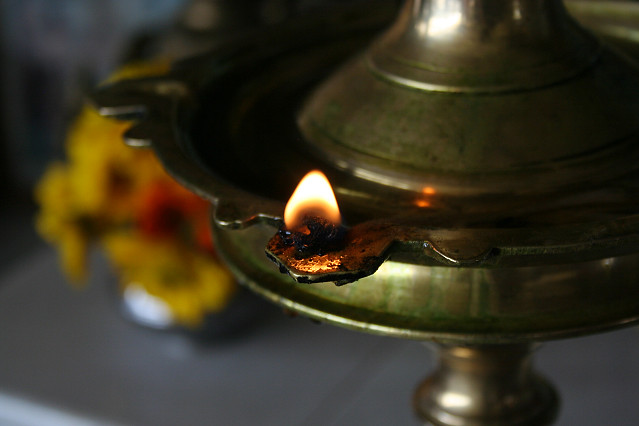This photo showcases a brass or copper decorative object, possibly an elaborate candle holder, set on a tabletop. The image is somewhat dark, making details slightly difficult to see. The main focus, occupying the right-hand side of the photo, is this intricately designed object which features a conical neck leading to a wider base. The object has a series of metal leaves or petal-like structures extending from its circular edge. A small yet vivid yellowish flame is emerging from one of these metal leaves, evoking the possibility of it being incense, a candle wick, or perhaps even flambe food. To the left of this central object, you can discern a tabletop with blurred elements, including a vase with yellow flowers resembling daisies and a single orange flower, although these elements are not in focus. The overall scene is dimly lit with the flame serving as the primary light source and visual focus amidst a muted, grayish background.